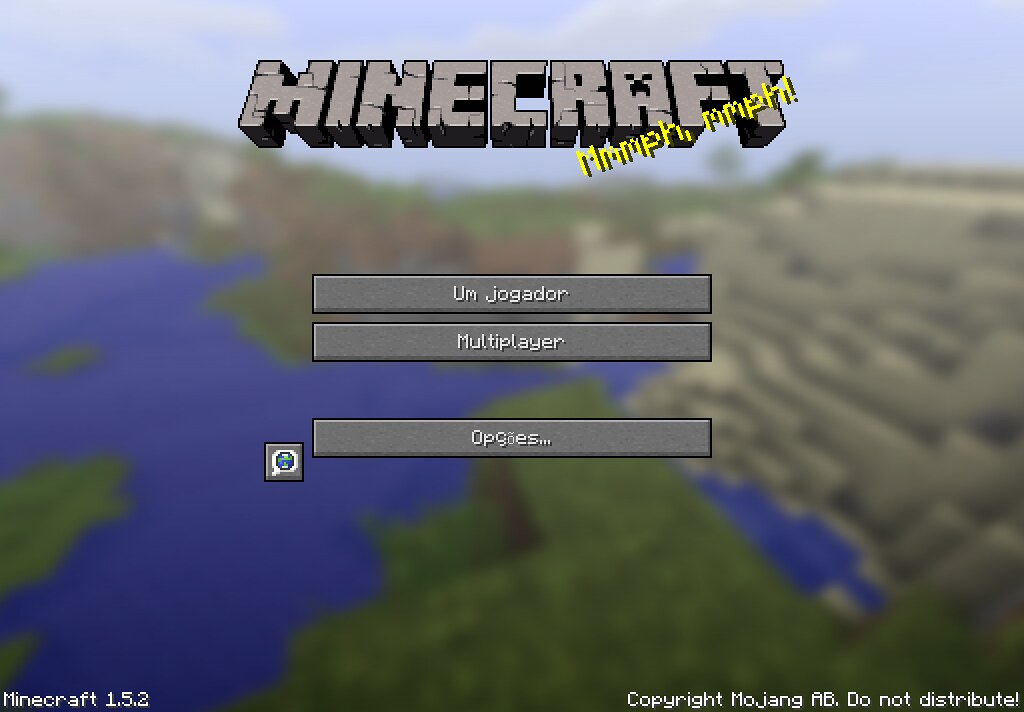The image shows the main menu screen of the computer game Minecraft 1.5.2. At the top center, the word "Minecraft" is prominently displayed in uppercase, slanted silver letters with a black shadow cast diagonally across the bottom right. A face is embedded within the letter 'A'. Across the letters, in a digitized yellow font, it reads "MMMPH, MMMPH!" Below the title, there are three long light gray rectangles bordered in black. The first rectangle displays the text "UM JOGADOR" in white, digital-like font, followed by "Multiplayer" in the second rectangle, and the third rectangle shows "Opções..." Left of the third rectangle is a small gray square bordered in black, with a speech bubble containing an image of the Earth inside it. The background depicts a blurry landscape featuring blue water, green areas, and some structures from the game. At the bottom, in white letters, it reads "Minecraft 1.5.2" and in the bottom right corner, "Copyright Mojang AB. Do not distribute."

This detailed caption was created by combining and refining aspects provided by multiple users, emphasizing common details to deliver a comprehensive description of the image.